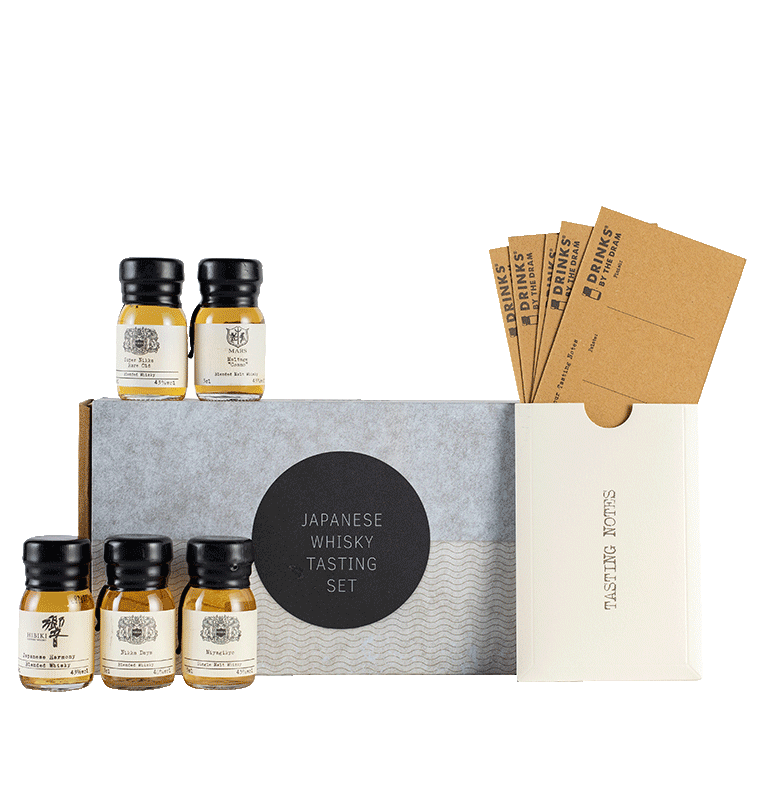This professional image, likely intended for a product advertisement, features a meticulously arranged Japanese whiskey tasting set against a pristine white background. At the center of the composition is a rectangular box, split into two designs: the upper half boasts a solid gray color resembling concrete, while the lower half displays a textured gray scalloped pattern. Prominently positioned in the middle of the box is a black circle containing the white text "Japanese Whiskey Tasting Set."

Surrounding the box are five whiskey bottles, each showcasing a transparent view of their amber contents. These bottles are capped with black seals and adorned with beige labels featuring various black logos, symbols, and text. Specifically, three bottles are aligned in front of the box, while two are placed on top.

To the right of the box, a cream-colored envelope labeled "Tasting Notes" is displayed upright. Additionally, there are brown note cards, made of a cardboard-like material, stamped with "Drinks by the Dram." These cards are presumably for users to jot down their tasting impressions. This carefully curated setup emphasizes the sophistication and thoroughness of the whiskey tasting experience offered by the set.